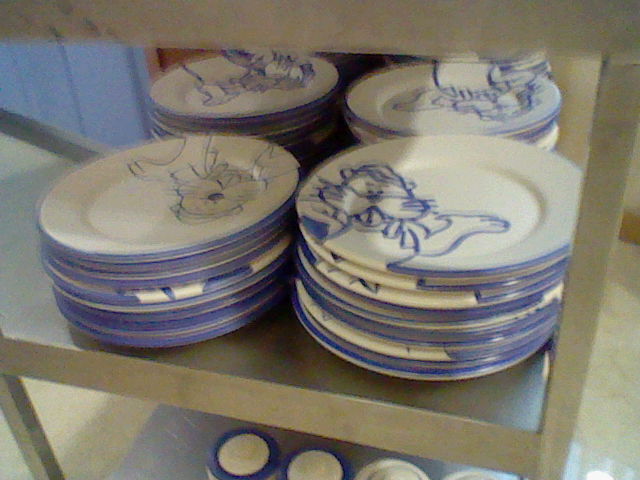A blurry and noisy photograph taken in a poorly-lit indoor setting captures a metal shelf laden with approximately 30 to 40 plates. Each plate, predominantly white with blue lines, displays unique cartoon figures, though the image quality makes the characters difficult to discern. The plate closest to the photographer features a cat. These plates, which may appear to be made of china rather than paper, are arranged on the top shelf of the metal rack. The image suggests a possible location such as a high school cafeteria, buffet, or hotel, with an additional, partially obscured second shelf beneath the plates, whose contents remain indeterminate due to the photograph’s blurriness.